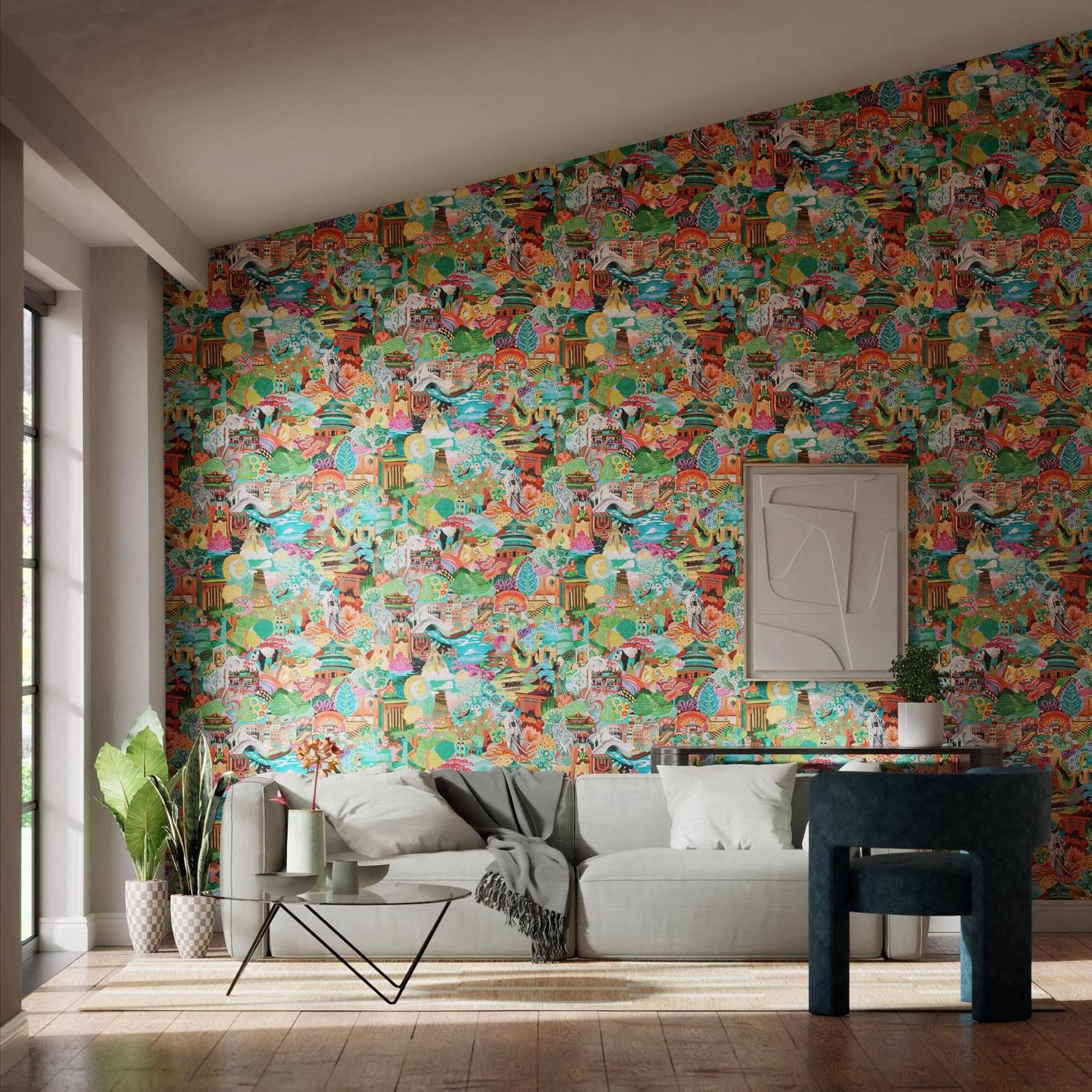This image depicts a meticulously arranged living room, seemingly designed for a magazine advertisement. Dominating the far wall is an intricate and vibrant wallpaper, possibly featuring an Asian-inspired print with prominent colors such as green, blue, pink, orange, and yellow, which seems to be the focal point of the room. The wall also hosts a framed modern art piece with a goldish-bronze frame and textured, off-white panels.

In front of the striking wallpaper, there is a long gray sofa adorned with two pillows – one white and one gray – and a matching gray throw blanket. A glass coffee table with black legs and a white candle sits to the left of the sofa, while a small black side table topped with a white pot containing a green plant stands by the sofa's right arm. Additionally, a dark green or blue velvet or microfiber chair enhances the room's luxurious aesthetic.

The left side of the image reveals part of a window, partially obscured by a white column, and two white plant pots containing upright green plants. Overall, the intricate details, from the window light to the various furnishings, contribute to a highly styled living room scene that prominently highlights the captivating wallpaper.